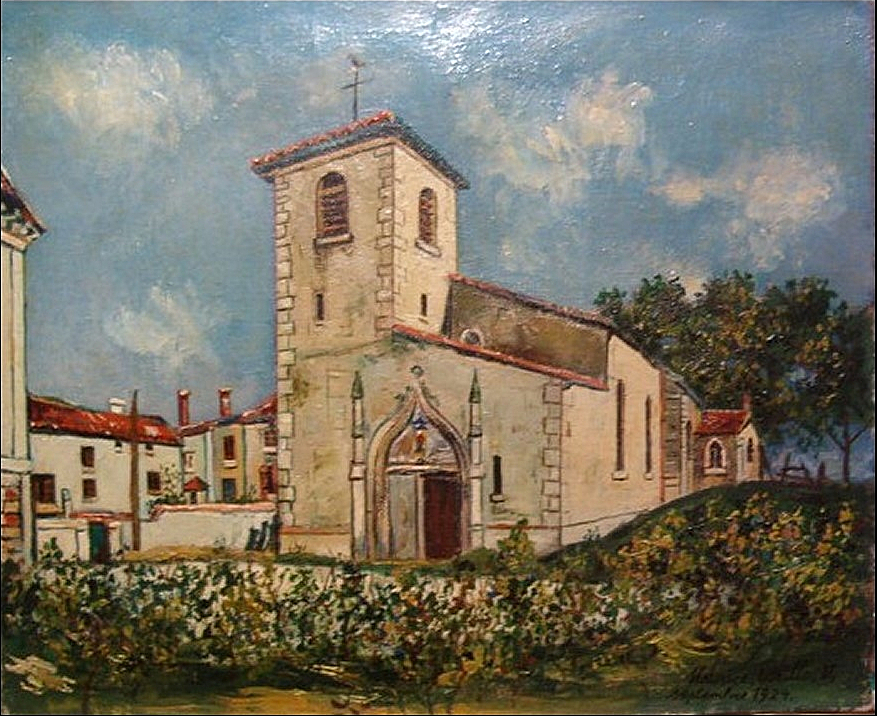The painting prominently features a white-stone church with a distinctive red roof, located in a verdant outdoor setting. The church’s most striking architectural feature is its square tower topped with a flat roof adorned with red shingles and a single cross. Arched windows and narrow rectangular slats punctuate the tower's walls. The church's main entrance boasts an ornate door, shaped like an Islamic arch that peaks at a narrow point.

Surrounding the church is lush greenery, with grass, plants, and hedges in shades of green, white, and yellow. To the left of the church, there is a courtyard alongside more stone buildings with red roofs. Behind the church are trees, contributing to the serene, natural backdrop.

The sky above is a vivid blue, scattered with patches of white clouds. The painting itself is shiny, especially noticeable in the upper area, and the artist's signature can be found in the bottom right corner. The scene evokes a South to Middle Eastern or Mediterranean ambiance, hinting at locations like Italy or Greece. This impressionist painting captures a tranquil moment with a beautifully structured missionary-style church at its heart.